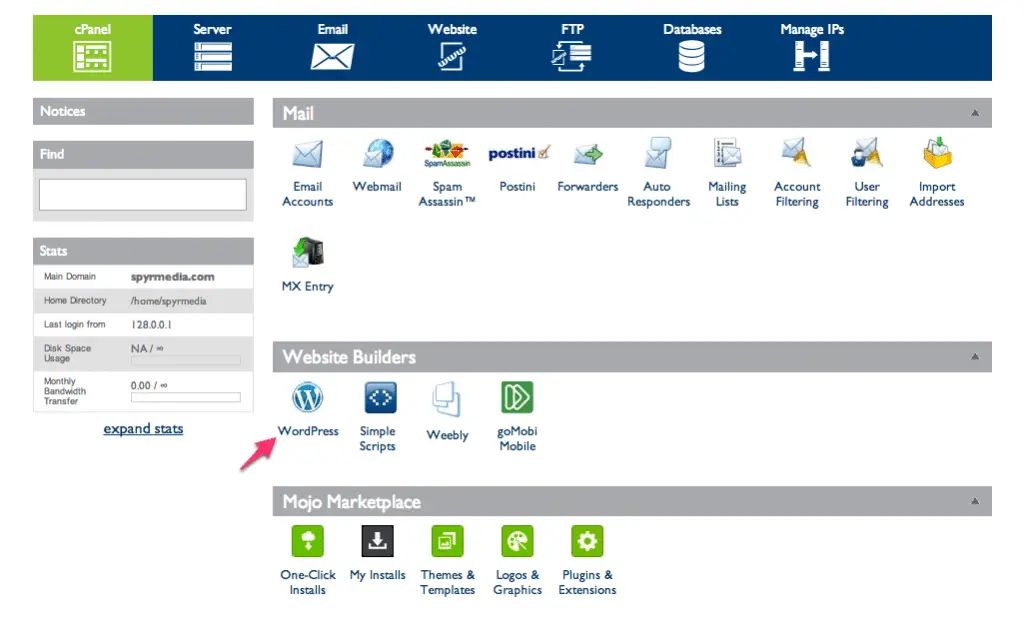This image depicts a computer screen displaying a program interface with a navigation bar stretching across the top. The navigation bar is blue, with a highlighted section on the left side distinguished by a green background. The green section features the word "cPanel" with a square icon beneath it. 

Adjacent to the green section, the blue navigation bar contains sequentially labeled tabs: "Server," "Email," "Website," "FTP," "Databases," and "Manage IPs." 

Below this navigation bar, the main content area of the screen features a predominantly white background. On the left side of this main section, there is a vertical column with gray segments, which include an empty white search bar situated beneath a header labeled "Find." Above the search bar, there is a section labeled "Notices."

Further down, the column lists various informational categories, such as "Stats," which is followed by details like "Main Domain," "Home Directory," "Last Login From," and "Disk Space Usage."

The right side of the page features a long gray bar labeled "Mail," which provides options for accessing different mail programs. Below this, there is a section dedicated to "Website Builders Programs," and underneath that, another section labeled "Mojo Marketplace."